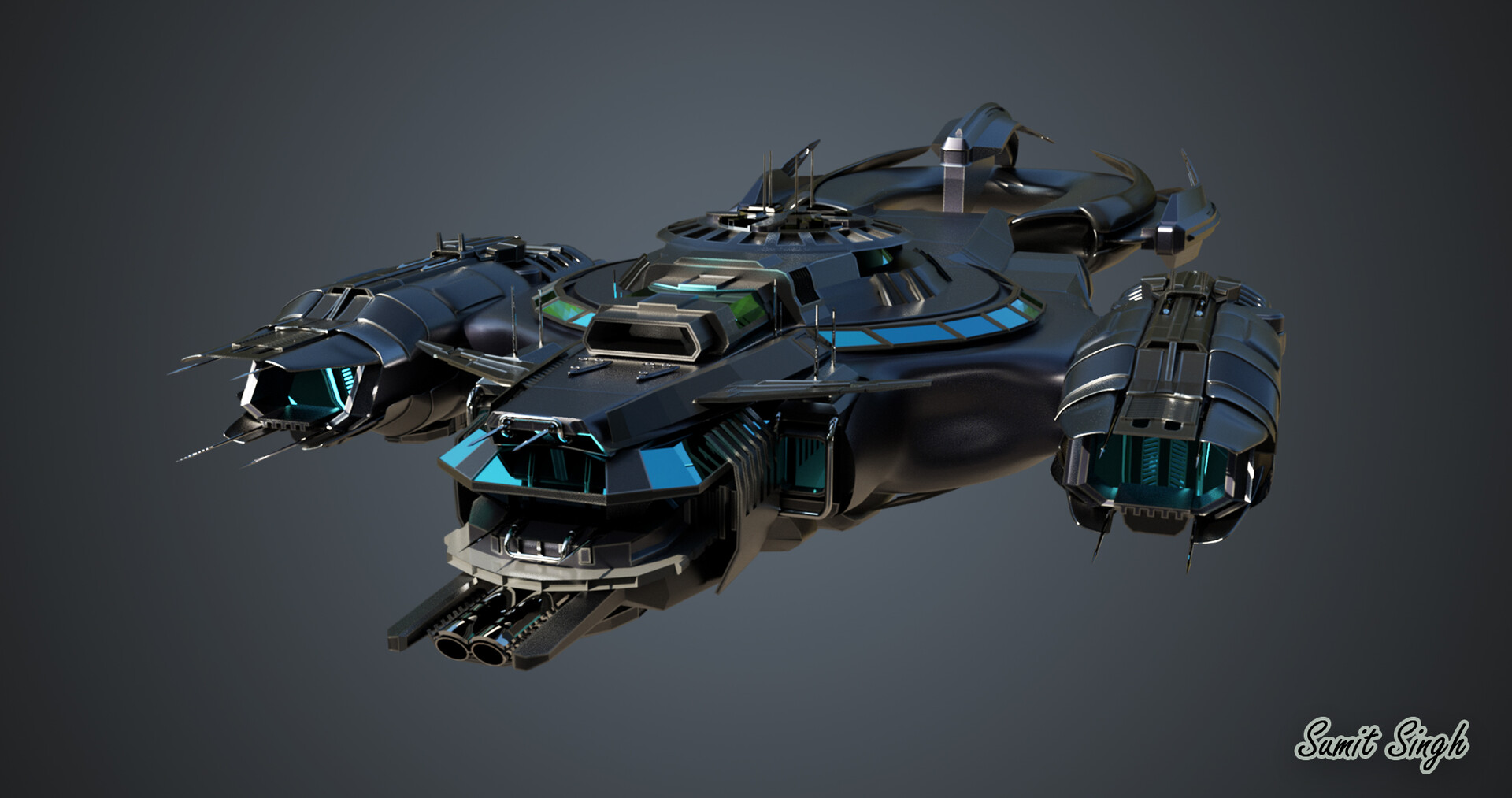This is a highly detailed 3D rendering of a massive, futuristic spaceship, complete with an intricate and textured design. The spacecraft features a primarily black hull with striking dark blue, green, and silver accents, and seems capable of housing a sizable crew. Notable for its imposing size, the ship includes a central core flanked by two narrowing corridors. The exterior is adorned with balconies and observation decks, adding to its advanced look.

The spacecraft's roof displays blue squares, contributing to its advanced aesthetic, while the engines on both sides showcase a fluorescent blue inner glow, suggesting powerful energy sources. Further embellishing the ship, blue rectangles arranged in a circular pattern can be seen atop the middle section. This complex visual is set against a dark gray background typical of rendering software, which lightens towards the middle, enhancing the spaceship's appearance. The image also features a watermark in the bottom right corner reading “SUMIT SINGH,” marking the artist's signature.